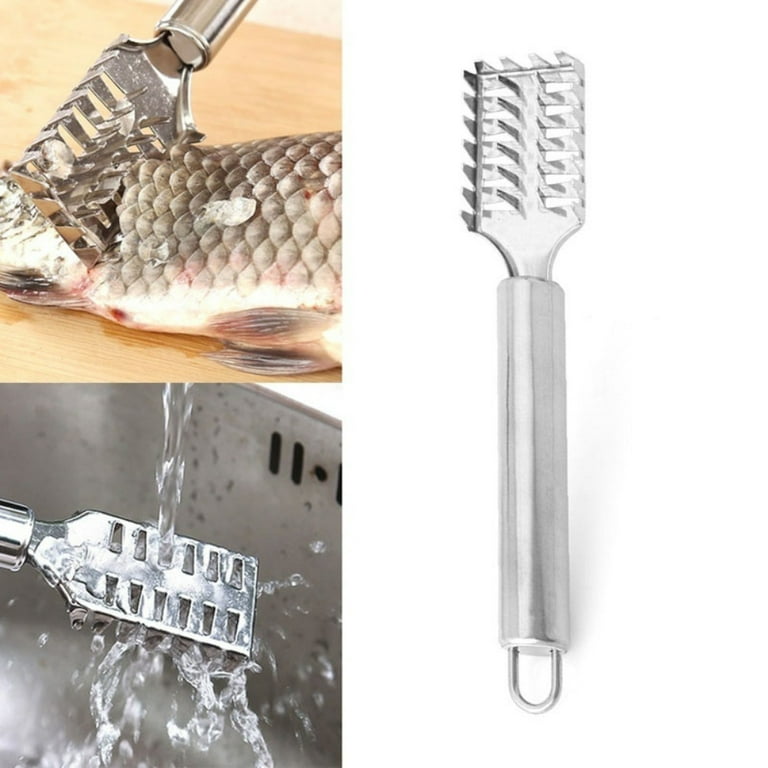In this composite image, which is divided into three different sections, various stages of using a fish scaling tool are meticulously depicted. The dominant element is a metal fish scraper, featuring a hand-sized handle and about 20 sharp blades aligned in a rectangular formation. In the upper left section, a person is actively using this tool to scrape off the scales of a fish, making it more suitable for human consumption. The tool's sharp teeth are being pressed against the fish's scales, efficiently removing them. In the lower left, the focus shifts to the cleaning process, where running water is being poured over the fish scraper to demonstrate its ease of washing post-use. The background colors span a spectrum from metallic gray and white to various shades of pink, red, and green, providing a vivid and detailed context for the activity taking place.